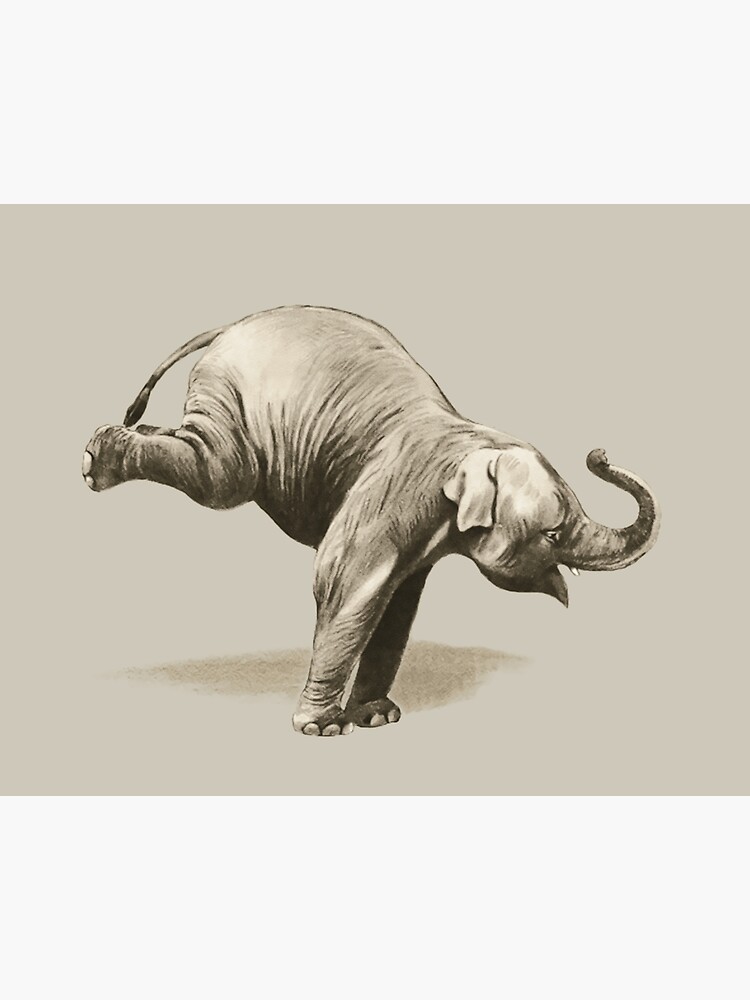The image showcases a detailed pencil sketch of an elephant balancing on its front legs with its hind legs extended straight behind it, almost parallel to the ground. The elephant is primarily light gray, with varied darker gray and black shading visible around its belly and rear, highlighting its textured skin with detailed wrinkles. The background is a soft gray, featuring shadowing beneath the elephant that enhances its three-dimensional appearance. Its trunk is gracefully arched above its head, curling forward, while its mouth is slightly open. The small tusks are depicted as almost inconspicuous, and its sad eyes are fixated towards the right side of the image. The elephant's ears are folded in on the sides of its head, and its tail extends outward with a noticeable thick black tuft at the end. The creature’s three toenails on each foot are clearly drawn, adding realism. Overall, the artwork captures the elephant in a dynamic pose suggestive of a dance or playful behavior.